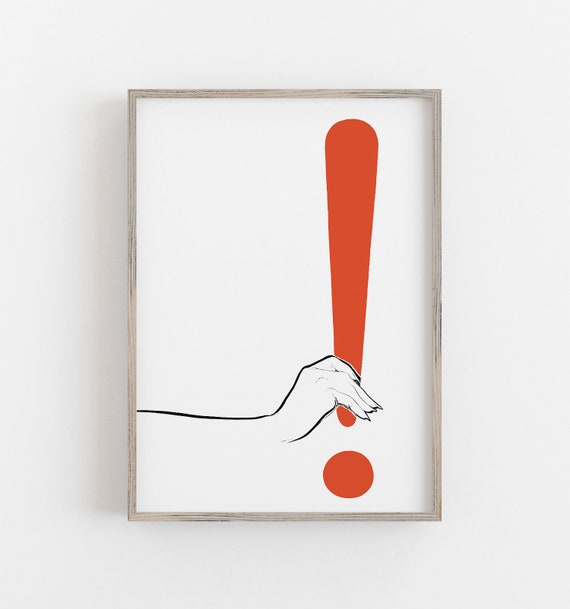The image depicts a large, rectangular painting displayed against a white wall, framed by a thin, light grayish border. At its center, on an all-white background, is a stylized, black and white outline of a human hand emanating from the bottom left and extending to the bottom middle. This hand, only partially drawn with sharp fingers and without a visible thumb, grips the bottom segment of a prominent red exclamation point. The exclamation point itself is positioned slightly to the right of the central vertical axis, extending from the bottom right towards the top right. The hand appears to pull the exclamation point slightly upwards, giving a subtle sense of motion. The artwork, with its minimalistic design and stark color contrasts featuring black, white, gray, and red, evokes a sense of playful abstraction, suggesting a piece that could be found in an art museum.